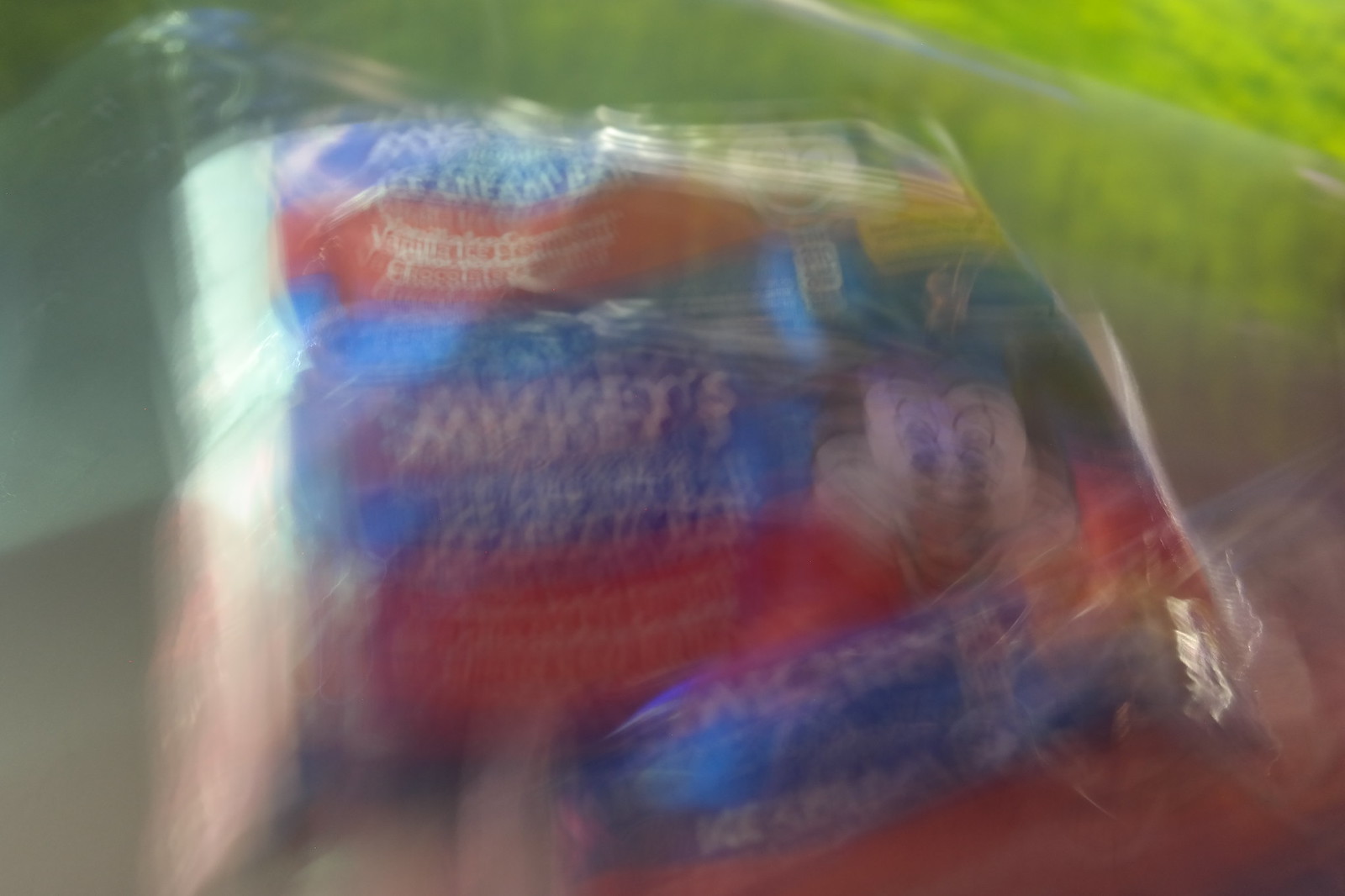The image depicts a highly blurred real-life photo of a flexible food package set against an outdoor backdrop with greenery, suggesting a tree or grass in the upper half and a red and grayish background at the bottom. The packaging appears crinkly and resembles a plastic bag commonly used for food products. The main focus is on the package, characterized by a white trim with alternating blue and red sections.

Dominating the package is the name "Mickey's," written in white text on a blue background, with additional white text on a red shape beneath it that remains unreadable due to extreme blurriness. There's an image of Mickey Mouse on the right side of the package, creating an optical illusion effect as if it's been duplicated or is in motion. The overall layout of the text and graphics suggests a rectangular food product, possibly an ice cream bar, but the blurred quality makes exact details indiscernible. The lower portion of the image shows an additional plastic bag lying on a glossy surface.